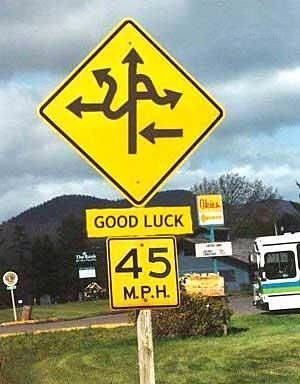The image depicts an outdoor setting captured in low quality and resolution, resulting in a somewhat blurry appearance. In the center of the frame stands a gray-colored pole supporting three signs. 

The top sign is diamond-shaped, adorned with a black border, and features five black arrows pointing in two different directions. Below it is a rectangular sign with a yellow background, bearing the text "Good Luck" in black letters. The bottom sign, also rectangular, simply displays the number "45."

Despite the poor image quality, the signs on the gray pole remain discernible, providing a focal point amidst the outdoors.